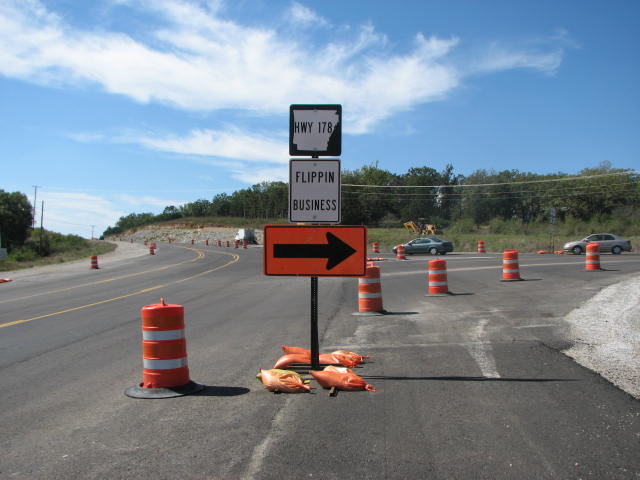The image depicts a clear, blue-skied day with scattered white clouds. It features a two-lane highway, designated as Highway 178, with a turning lane in the middle outlined by yellow lines. The focal point is a state sign indicating "Highway 178" situated above a sign that reads "Flippin' Business". The Highway 178 designation is in black on a white state symbol, while "Flippin' Business" is in black housed within a white sign bordered by black. Below these signs is an orange detour sign with a black arrow directing traffic to the right. The road is undergoing maintenance, indicated by orange and white striped barrels and cones that block the path and guide vehicles toward the detour. There are a few cars visible in the background near the intersection, moving to the left, while a dump truck or similar type of tractor is parked on the grassy area nearby, surrounded by trees and power line poles. The scene suggests a redirection for reaching local businesses during the roadwork.